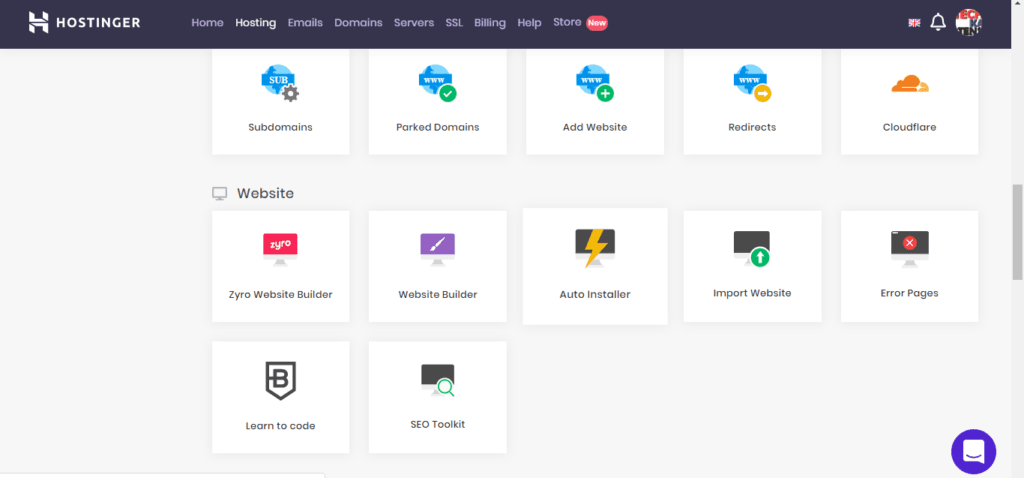A screenshot of the Hostinger webpage is depicted, showcasing its comprehensive dashboard and user interface. The webpage header features the Hostinger logo, characterized by a stylized "H" icon. The navigation bar at the top lists various tabs including Home, Hosting, Emails, Domains, Servers, SSI, Billing, Help, and Store. To the far right, a bell icon, followed by another unclear icon, is visible.

Beneath the header, the dashboard is organized into 12 sections, each presented as square tiles with distinct icons and labels. The top row includes Subdomains, represented by a blue earth icon accompanied by a small gear; Park Domains and Add Website, both sharing the same blue icon; Redirects with the same blue earth icon; and Cloud Store, distinguished by an orange cloud icon. 

The second row, under the subheader "Website," contains the following: Zyro Website Builder, identified by a red computer monitor icon; Website Builder, with a purple rectangle and a white pen icon; Auto Installer, marked by a monitor with a yellow lightning bolt; Import Website, denoted by a computer monitor with a green arrow; Error Pages, featuring a monitor with a red X; Learn to Code, shown with a shield icon bearing a "B"; and SEO Toolkit, again with a monitor icon.

In the bottom right corner, a purple circle, likely a chat button, completes the interface layout, indicating user support availability.